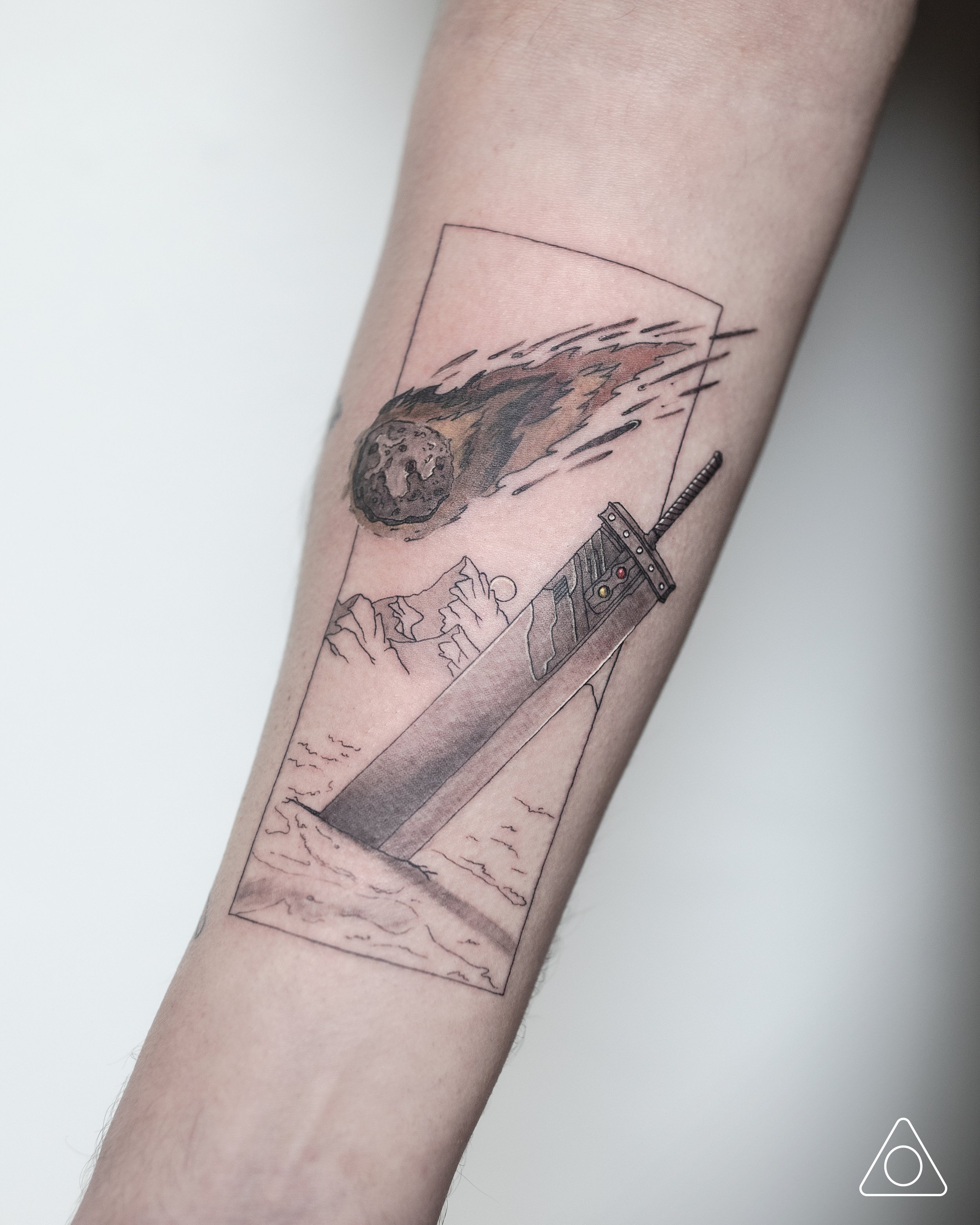The image depicts a detailed tattoo on a Caucasian individual's forearm, set against a grayish off-white background that darkens towards the right. In the bottom right-hand corner, there's a small logo consisting of a white-line triangle with a circle inside it. The tattoo is framed within a thin rectangular border and contains several distinct elements. 

At the top of the tattoo, a black and tan comet or meteor with trailing orange flames is angled downward as if descending from the sky. Below the comet, a mountain range is featured with either the moon or sun rising or setting behind it. The ground below the mountains is textured, and implanted in this ground is a large, rectangular-bladed sword or dagger with a small handle, presenting a metallic, silver appearance. The sword also features a circular embellishment with red and yellow accents, adding a futuristic flair to the overall monochromatic scheme of the tattoo.